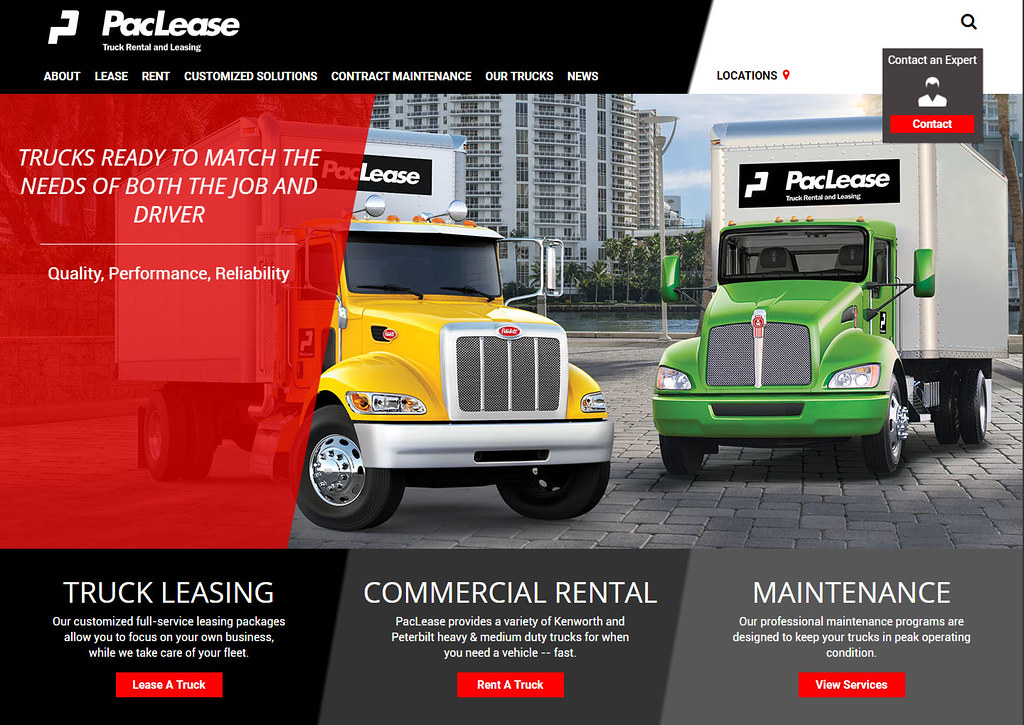**Detailed Description of PackLeash Website Homepage:**

The homepage of PackLeash, a truck rental and leasing company, is prominently displayed with a sleek and professional design.  

In the **top left-hand corner**, the PackLeash logo and name are prominently positioned on a **black panel**. Directly beneath the logo, there's a navigation menu featuring various headings such as **"About," "Leash," "Rent," "Customized Solutions," "Contract Maintenance," "Our Trucks," and "Use."** 

On the **right-hand side**, set against a white backdrop, there's a **"Locations" link** and a **red "Contact" button** housed in a drop-down menu. This section is designed for users to get in touch with an expert for further assistance. Additionally, a small **search icon** is visible in the top right-hand corner for easy navigation.

Below the navigation area, the content is divided into visually distinct sections. A central image showcases **two trucks**—one yellow and one green—positioned prominently on the page. To the left of this central image, a **red banner** occupies about a third of the screen, displaying the text: **"Trucks ready to match the needs of both the job and driver."** Below this are the words **"Quality, Performance, Reliability"** etched clearly.

Along the base of the screen, three distinct sections align horizontally: 
1. A **black panel** covering truck leasing, accompanied by a **red button labeled "Leash a Truck"**.
2. A section entitled **"Commercial Rental"** with a **red button labeled "Rent a Truck"**.
3. A **light gray panel** that details **maintenance services**, featuring a **red button labeled "View Services."**

Every element of the homepage is meticulously organized, guiding users to easily access the services and information they require.